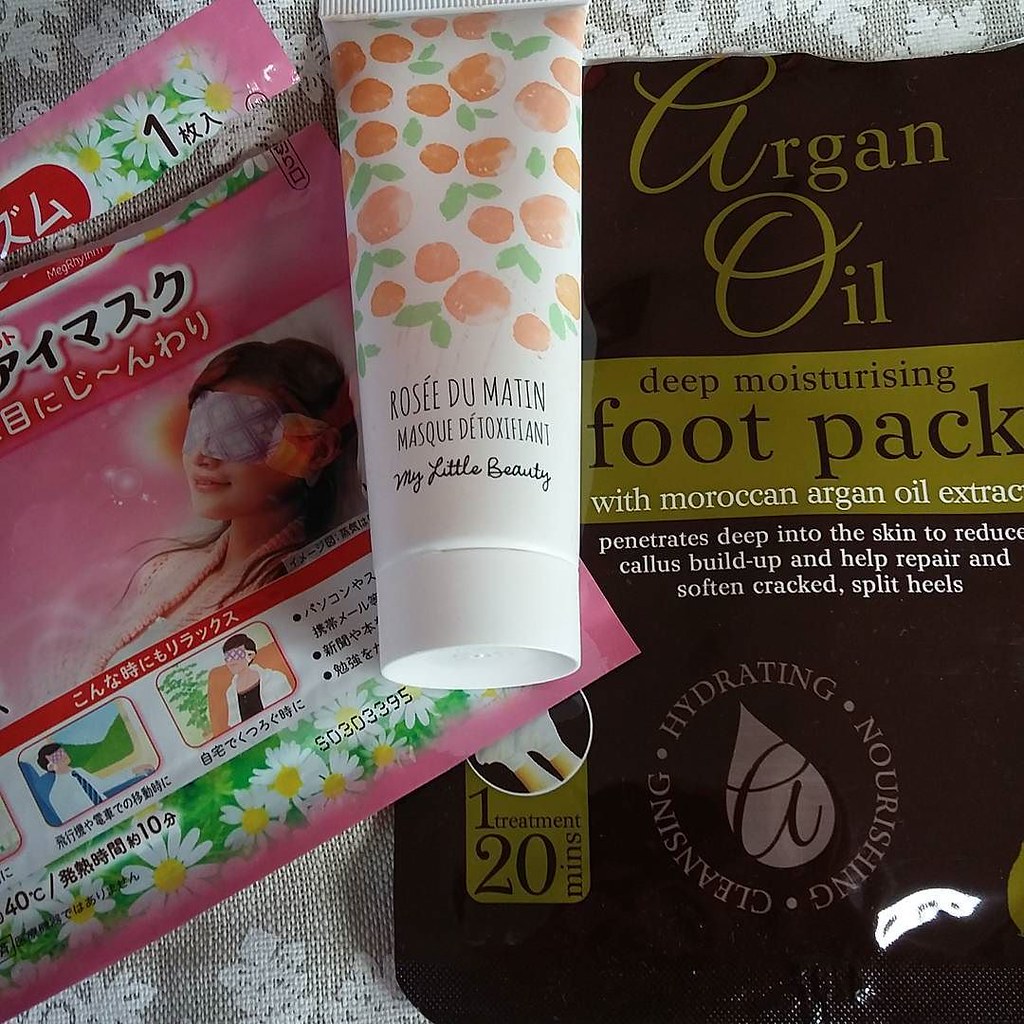The photograph depicts a skin care collection artfully arranged on a delicate piece of white lace fabric. The display features three distinct items. 

To the left, a torn pink packaging reveals what appears to be a Korean eye mask with the top slightly ajar and partially separated from the bottom. The packaging showcases an illustration of a woman lying down, wearing a gray mask over her eyes. The text, which is mostly in Korean, is accompanied by an image of white daisies set against a green background.

In the center lies a white tube adorned with illustrations of peaches complete with green leaves. The text on the tube reads "Rosé du Maine, Matin, Masqué des Fonts, My Little Beauty." This tube features a white cap at its base.

On the right side of the composition, a black package presents itself as a foot mask enriched with argan oil. A prominent gold banner proclaims it as a "Deep Moisturizing Foot Pack with Moroccan Argan Oil Extract." Detailed text on the packaging promises that the foot pack "penetrates deep into the skin to reduce callus build-up and help repair and soften cracked split heels." An additional teardrop icon emphasizes the benefits by listing "hydrating, nourishing, cleansing."

Each element of the image is meticulously positioned, creating an inviting and elegant presentation of these skincare products.